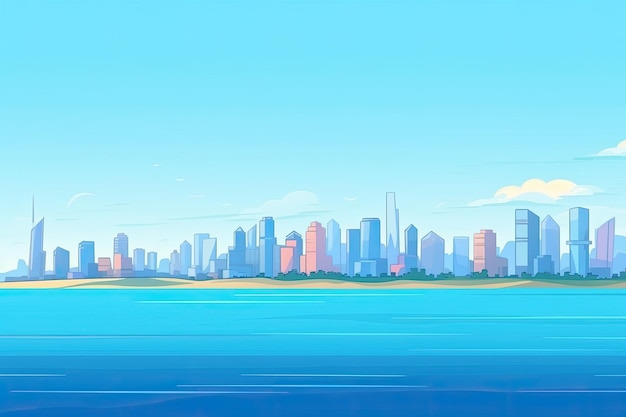The image is an animated illustration of a distant cityscape, portrayed in a quasi-cartoonish style. Dominating the foreground is a vast expanse of sea that transitions from a bright to a darker blue as it moves downward in the image, with subtle white lines suggesting waves. A narrow strip of sandy beach lies just above the water, complemented by patches of greenery with a few trees. Beyond the beach, numerous skyscrapers and high-rise buildings populate the skyline, painted in hues of red, beige, light blue, gray, pink, and predominantly blue, which harmonize with the colors of the sea and sky. The sky itself is a light blue, lighter than the sea, scattered with a few puffy white clouds, and white lines to indicate wind. The scene is tranquil and devoid of any human presence or textual elements, creating a serene urban landscape.